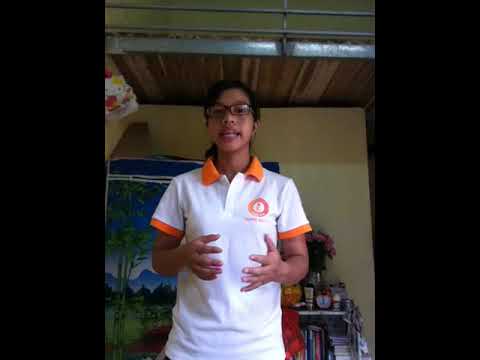A young boy with medium skin and black hair parted to the left is standing facing the camera from the waist up. He is wearing a white short sleeve shirt with an orange collar and orange trim just above the elbows. The shirt also has an orange emblem on the chest. Both of his hands are held straight forward, almost touching, as if he is holding an invisible ball, and his mouth is open, revealing both rows of teeth, suggesting he is talking. He is wearing large eyeglasses with a slight reflection on one lens. Behind him is a yellow wall, a wooden platform with a metal railing on top, and a banner depicting a blue sky with green trees, green grass, and blue mountains. To the right of him, there is a shelf with various objects on it, including jars, bottles, and flowers. The ceiling above has wood planks.